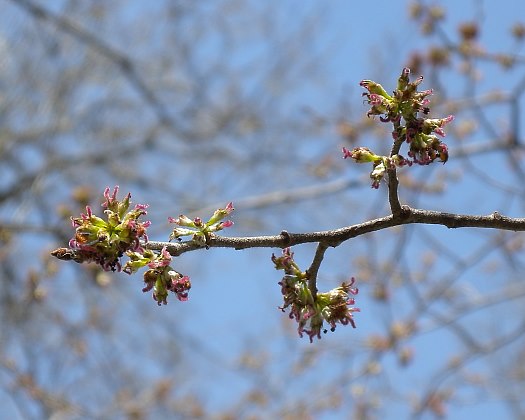In this close-up nature shot taken during the daytime in springtime, a single tree branch in the foreground takes center stage. The branch is brown and adorned with vibrant green leaves and budding flowers that exhibit a blend of light purple, green, and pinkish tips—potentially indicating the future blossom color. The blossoms seem to cluster along the right side, transitioning smoothly toward the left. The background features a beautiful blue sky and additional branches, though these elements remain blurred, creating a bokeh effect that keeps the focus firmly on the flowering branch. The overall composition showcases the delicate, emerging beauty of nature in spring.